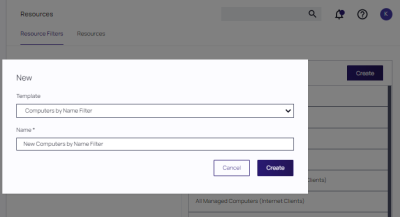The image depicts a small, detailed interface, likely part of an IT management system used by administrators to manage network computers. The interface consists of two main layers. 

The background layer displays a resource page titled "All Managed Computers" and features a search bar at the top right alongside icons for notifications, user profile, and help (indicated by a question mark). The background hues are predominantly white, providing a clean and professional appearance.

In the foreground, a pop-up window titled "New" prompts the user to select a template and provide a name. The default template is set to "Computers by Name Filter," and the default name matches this template. The pop-up includes options to either cancel or proceed with the creation process—the latter signified by a hard-to-see purplish-blue "Create" button. However, the purpose and specifics of what is being created or what the filters entail remain unclear due to the lack of additional contextual information.

Overall, the image appears to be part of an administrative interface designed for managing networked computers, likely used by IT professionals.